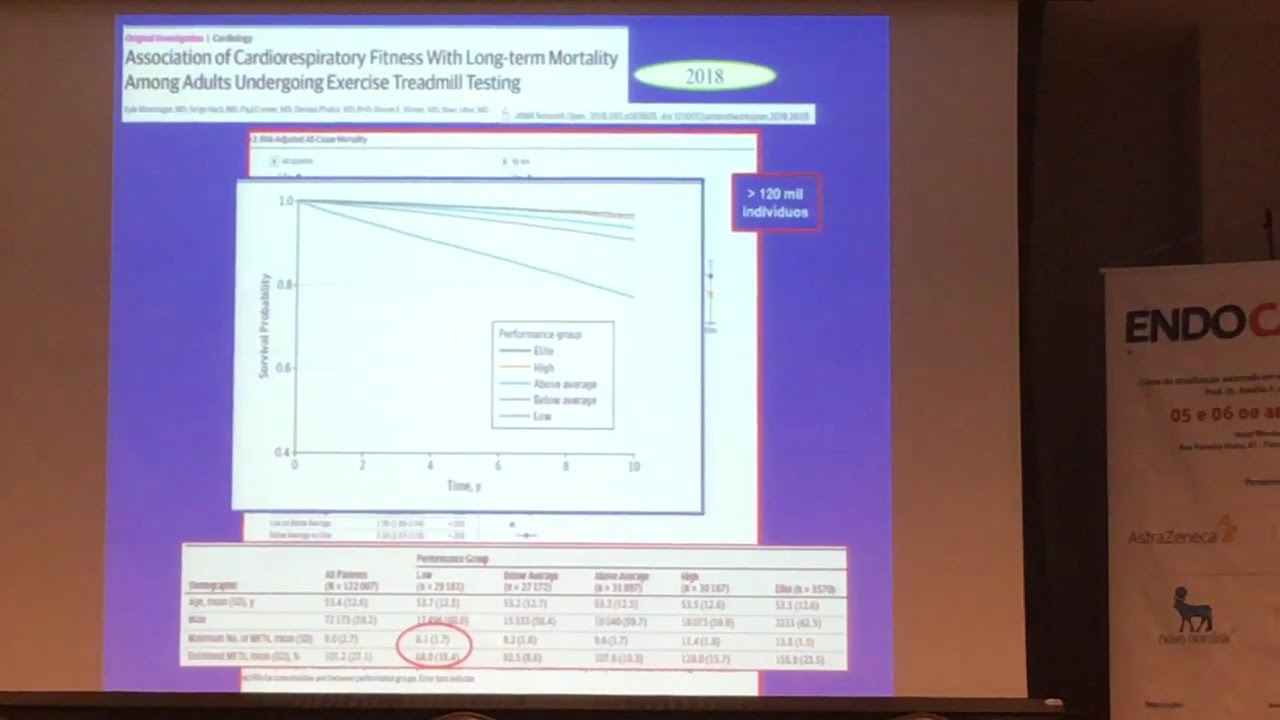The image depicts a photo of a projector screen displaying a PowerPoint slide from a 2018 presentation. The slide's title, "Association of Cardiorespiratory Fitness with Long-Term Mortality Among Adults Undergoing Exercise Treadmill Testing," is prominently shown in a white box in the top left. To the right of the title, an oval bubble indicates the year "2018." Below the title, a graph charts survival probability on the y-axis (with values 0.4, 0.6, 0.8, and 1.0) over time on the x-axis (marked 0, 2, 4, 6, 8, and 10 years). The graph's curves are color-coded and labeled as elite, high, above average, below average, and low, illustrating varying levels of cardiorespiratory fitness. Additionally, there's a table with text and data at the slide's bottom. The image has red borders around sections, including a red box in the top right with an arrow and “120 mil individuos” in white. On the right side, a freestanding stand displays logos, including AstraZeneca and Nordisk, with text reading "endo" in black. The background is a purple template with various charts and graphs, although the details are partially obscured due to poor lighting and a blurry image. No people are visible in the image.